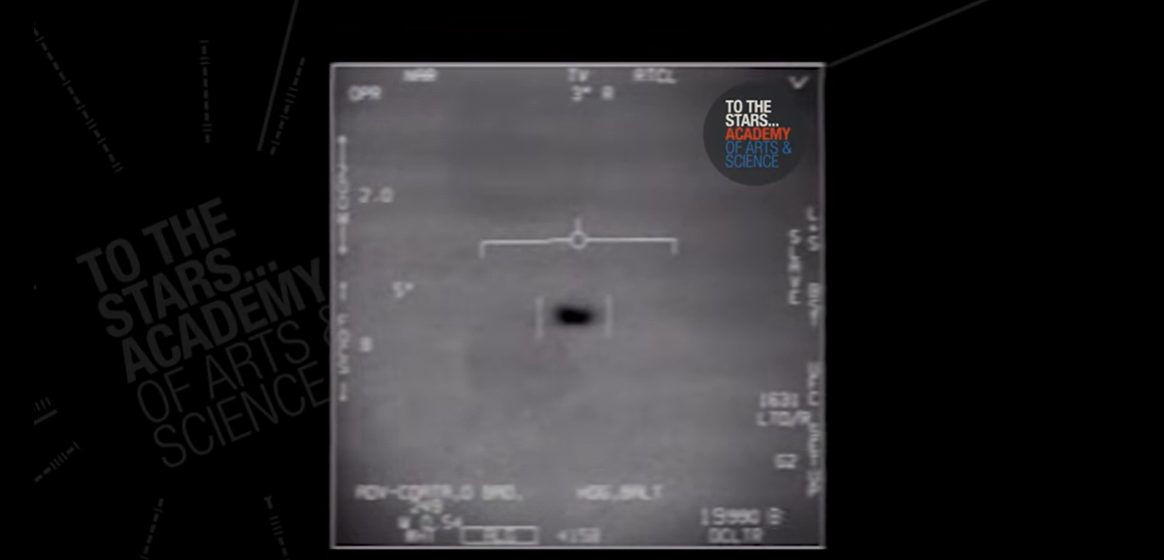The image features a blurred grayscale square set against a black background, reminiscent of surveillance or possibly scientific instrumentation. At the forefront, within the square, a prominent black dot sits centrally, surrounded by faint, nearly illegible text and undistinguishable numbers and letters scattered around the perimeter. Above the dot, white lines seem to measure the dot itself. The upper right corner of this gray square contains a circular label adorned with multi-colored text—white, red, and blue—reading, "To the STARS Academy of Arts and Science." Additionally, outside the square to the left, similar text appears in the black background, though in a more muted gray font. This cryptic, grainy image evokes the imagery often associated with UFO photography or high-altitude surveillance, and its connection to the STARS Academy hints at a scientific or exploratory purpose.